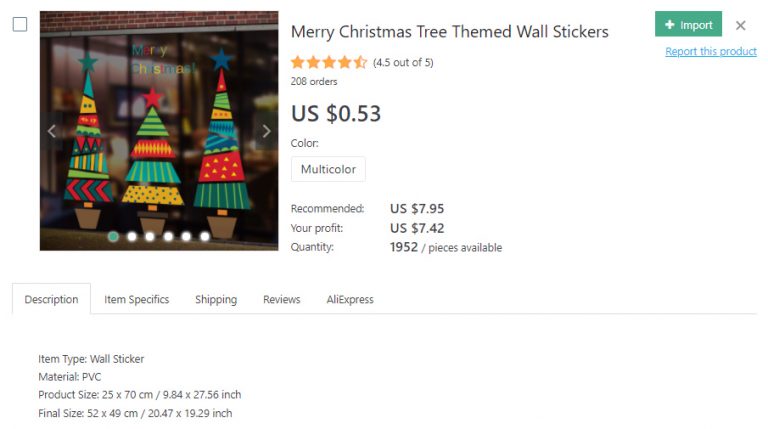**Image Caption:**

The thumbnail features a vibrant display of Christmas-themed wall stickers, showcasing a festive "Merry Christmas" message with a tree motif. Rated at an impressive 4.5 stars out of 5, these stickers have garnered a total of 208 orders within the U.S. The price is an attractive 53 cents per unit. 

The image includes three eye-catching, geometric Christmas trees in assorted colors. The tree on the left is adorned with a blue star at the top and decorated with blue, yellow, red, and green shapes, including arrows. The middle tree features segments of green with stripes, red, and blue interspersed with confetti-like yellow sections. The third tree follows a similar style. Surrounding the trees is a series of white dots, adding a snowy festive touch.

To the right of the image, a recommendation banner suggests a profit margin for resellers, indicating a potential profit of $7.42 from a sale price of $7.95. It also highlights an available stock of 1,952 pieces.

Below the thumbnail, an open description tab provides detailed product information, including the material composition, item type, product size, and final size. Additional tabs offer specifics on shipping, customer reviews, and the source, Aliexpress. This image serves both as an enticing display for potential buyers and an informative tool for resellers.